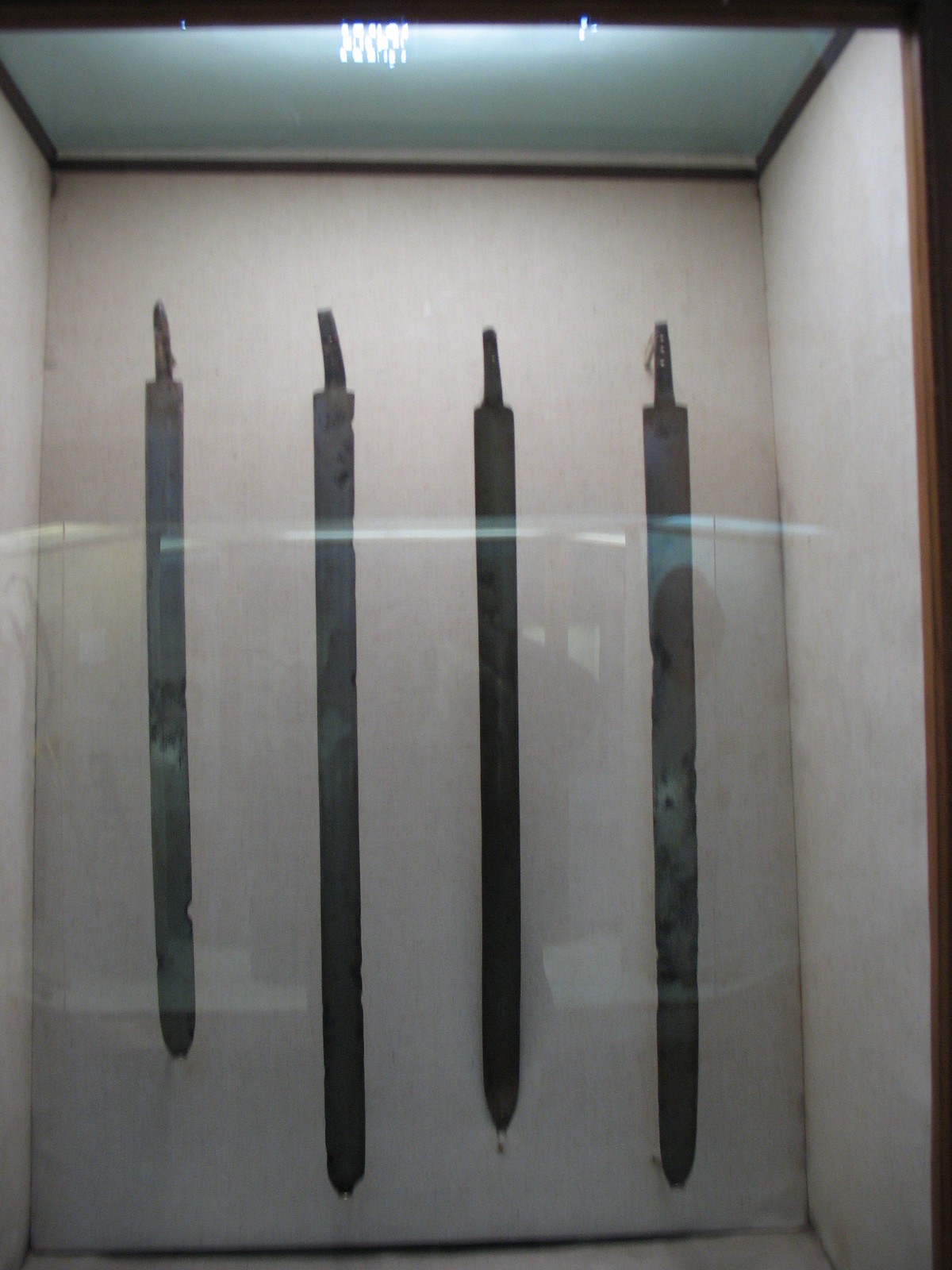The image displays a square, white wooden display case with a glass front, illuminated by light from the top. Inside the case, set against a beige backdrop, are four ancient swords, each sheathed in black. The swords have long, darkened blades with short, slender black handles, which feature intricate engravings or letters. Reflections on the glass front and the surrounding white frame are visible, adding to the display's illuminated and pristine appearance.